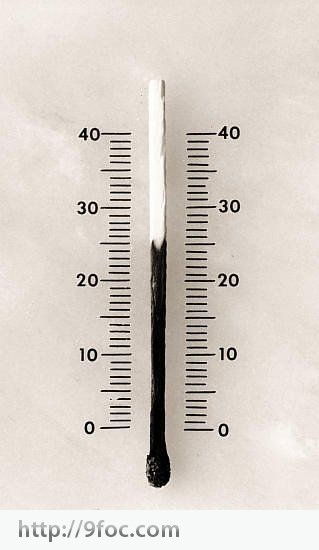This intriguing image features a vertical, rectangular, white background resembling a piece of paper. In the center of this background is an inventive representation of a thermometer. However, instead of a traditional glass tube with red mercury, the thermometer is creatively depicted using a wooden matchstick. 

The matchstick is oriented vertically with its unburnt, sulfur-tipped end pointing downwards. The burnt portion of the match extends upwards, visually representing the mercury. The charring on the match stops at the 25 mark on a scale that ranges from 0 to 40 on both the left and right sides of the image.

At the top, the burnt match head symbolizes the bulb at the bottom of a conventional mercury thermometer. The matchstick's charred portion gradually transitions to unburnt wood, suggesting a clever visual analogy of a temperature rise. Additionally, a watermark reading "http://9foc.com" is placed across the bottom of the image.

This clever artistic rendition captures the essence of a thermometer using a common household item, highlighting creative innovation through simple design elements.